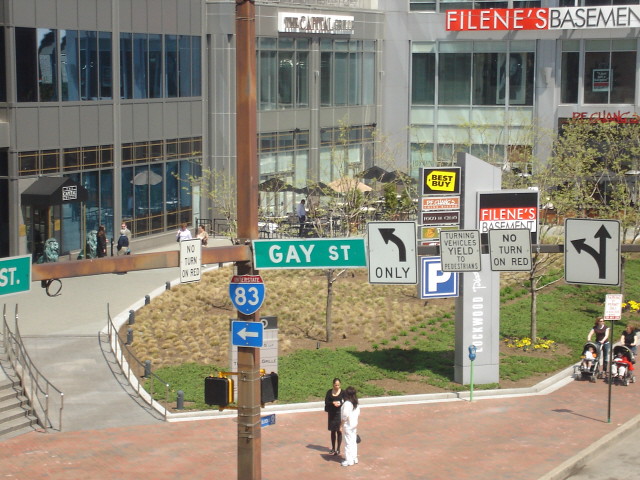The photograph captures a bustling courtyard area in front of a contemporary office building with ample windows. In the center of the image, there is a circular patch of green grass sided by short, round vegetation, which is surrounded by both a red brick sidewalk and a gray asphalt sidewalk. On the red brick path, two women, one dressed in white and the other in black, stand beside a metal pole engaging in conversation. The pole holds several street signs, including a green one that reads "Gay Street," an interstate sign for Route 83 with a left-pointing arrow, and a white "No Turn on Red" sign. Additionally, there is a blue arrow and walk/no-walk signal boxes on the pole. Nearby, two more women push toddlers in strollers past a parking meter and several other road signs. Storefronts for Filene's Basement, Best Buy, and P.F. Chang's are visible, with Filene's Basement and P.F. Chang's signs prominently displayed on the building in the background. The building also features a few tables with umbrellas out front, adding to the vibrant, multi-purpose character of the district.